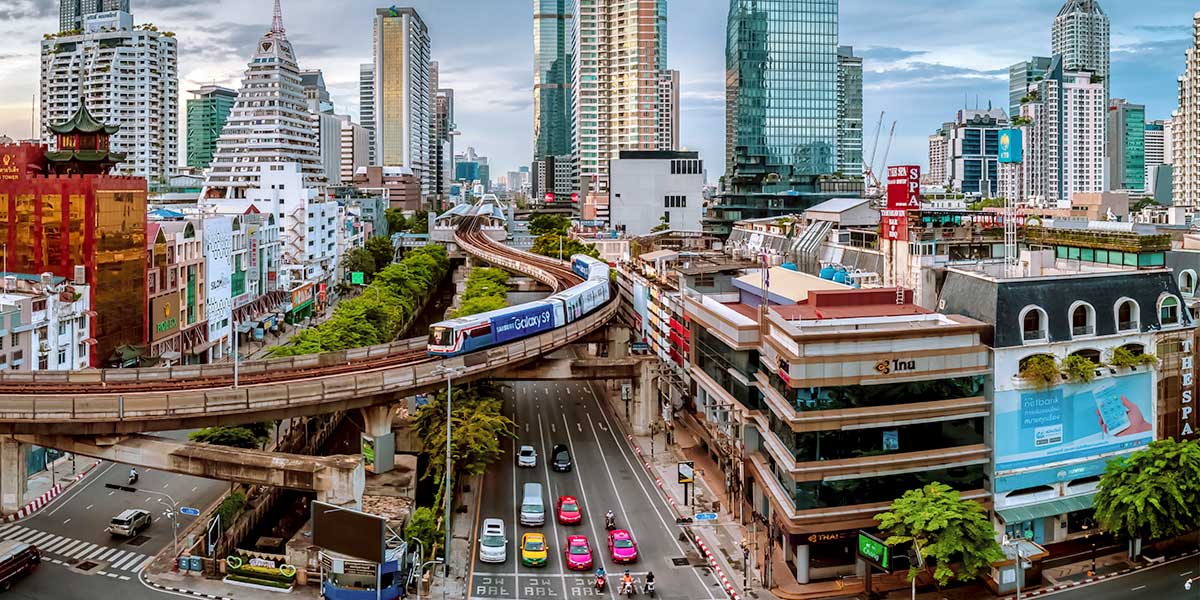This aerial photograph, likely taken from around 100 feet above ground level, captures a bustling, possibly Asian city during the day, with a vivid blue sky dotted by gray clouds. Dominating the middle of the image is a raised train platform, with a blue and white train displaying an advertisement for the Galaxy S9 against a blue background. Below the tracks, a five-lane road teems with traffic, including two purple cars, a red car, a yellow car, a white car, and a white truck. The urban landscape showcases an eclectic mix of architecture, including towering skyscrapers with metallic facades, some featuring triangular shapes and extensive glass exteriors. An advertisement depicting a cell phone and hand is prominent on one building, while others display various company symbols and signage such as "ING" and a vertically oriented "Spa." Interspersed among this concrete jungle, patches of greenery and trees add contrast to the scene, though the exact location of the city remains undetermined.